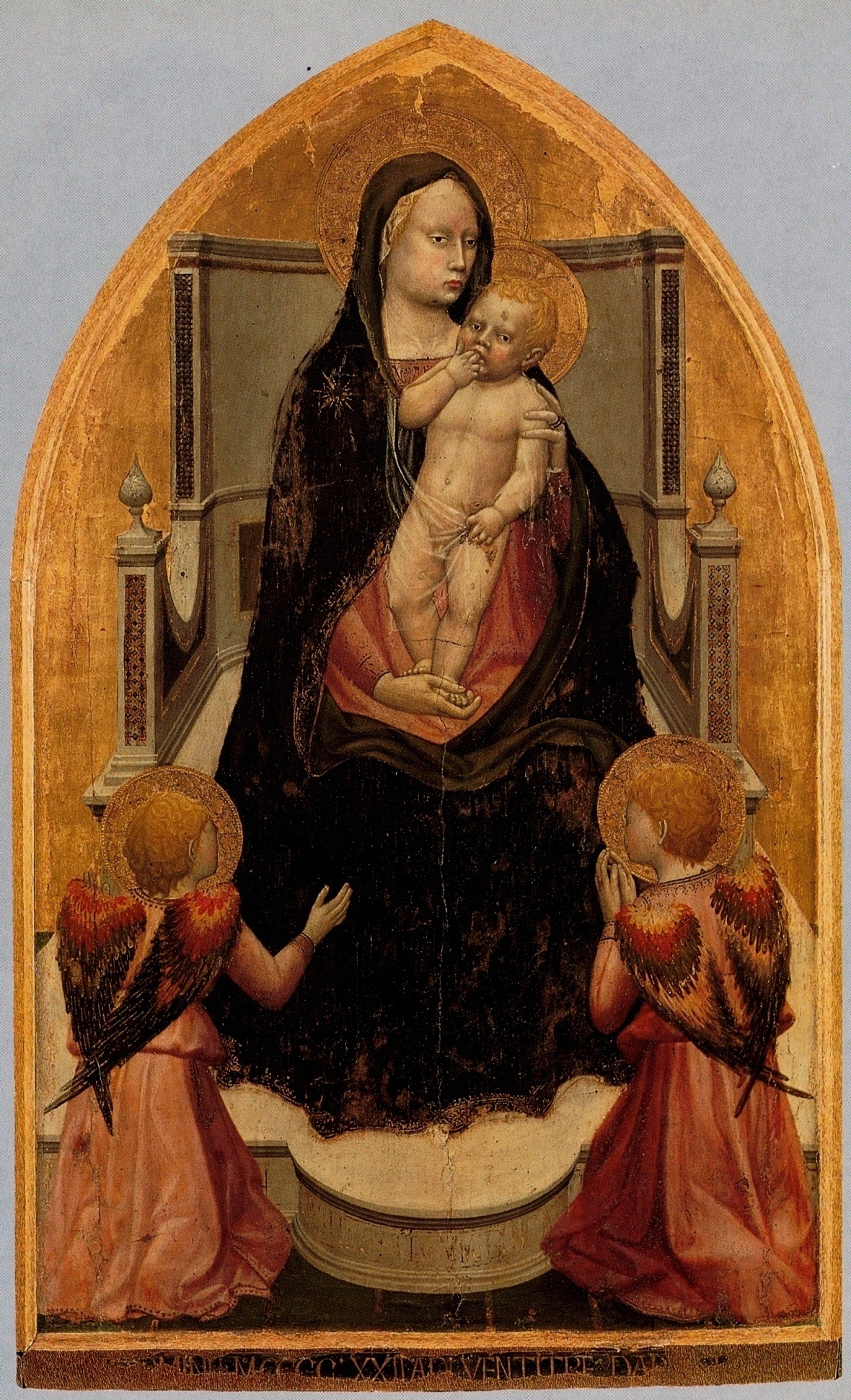The painting appears to be a Renaissance-style depiction of the Virgin Mary and baby Jesus. Mary is seated on a stone throne, adorned in a pinkish-red shirt under a black shawl, with intricate patterns visible on her garment. She has blonde hair and is looking sideways, lovingly embracing Jesus. Jesus, also blonde and with a halo, is standing on her lap with two fingers in his mouth and is holding a piece of cloth to cover his private parts with his other hand. His tiny feet rest in his mother's right hand, while she supports his left shoulder with her left hand. Both mother and child are encircled by golden halos.

Flanking Mary are two small angels, each with haloes around their blonde heads and richly colored wings in shades of reddish-black and pink. The angel to the left is shown with open hands, while the angel on the right is depicted in a praying stance with hands folded. The angels wear pinkish-red garments and kneel at her feet on either side of the raised, patterned platform upon which Mary rests her feet. The background of the painting radiates a tannish-gold hue, giving the scene a celestial ambiance. The throne Mary sits upon and the platform at her feet suggest a sense of reverence and sanctity, typical of the Renaissance era's artistic focus on religious iconography.